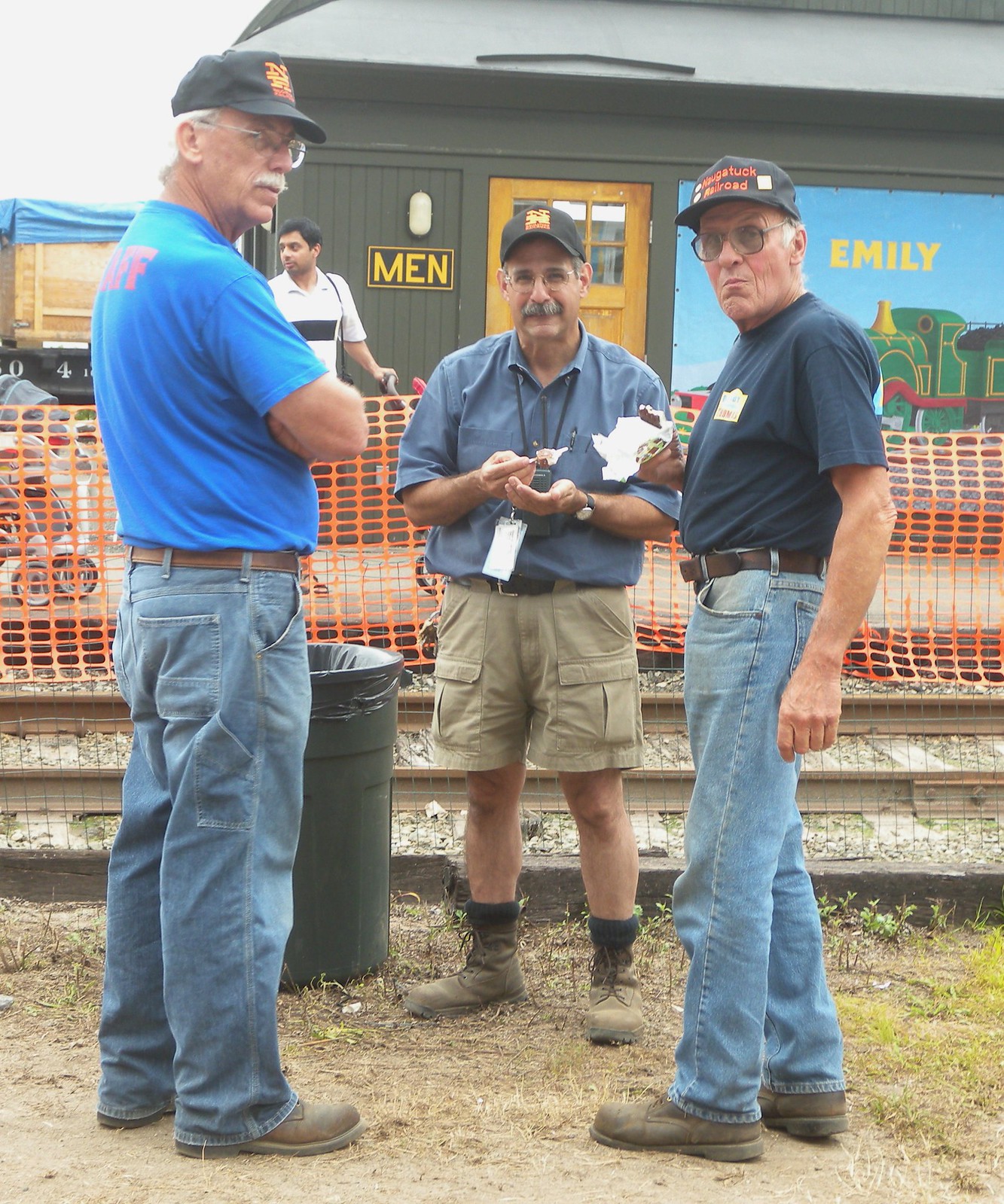In this image, three elderly men, likely in their 60s or 70s, are posing for a picture and staring at the camera. They are all wearing black baseball caps and casual attire: the man on the left is in blue jeans, a blue shirt, and a black cap; the middle man is dressed in cargo shorts, a dress collared blue shirt, some light brown boots, and a lanyard around his neck; the man on the right is in dark blue jeans, a dark blue shirt, and light brown boots. All three men wear brown belts.

They are eating ice cream sandwiches, with two of them actively holding the treats. The men are gathered near a trash can on the right side, standing on a patch of dirt with a little grass, next to some railroad tracks.

In the background, there is a building with dark green walls. This building has a wooden door marked with a yellow sign that says "MEN," likely indicating a bathroom. There is also yellow text on the green wall that reads "EMILY." Additionally, a man with a white collared t-shirt featuring a vertical black stripe can be seen faintly in the background. The building has a train design painted on it, contributing to the ambiance of the scene.